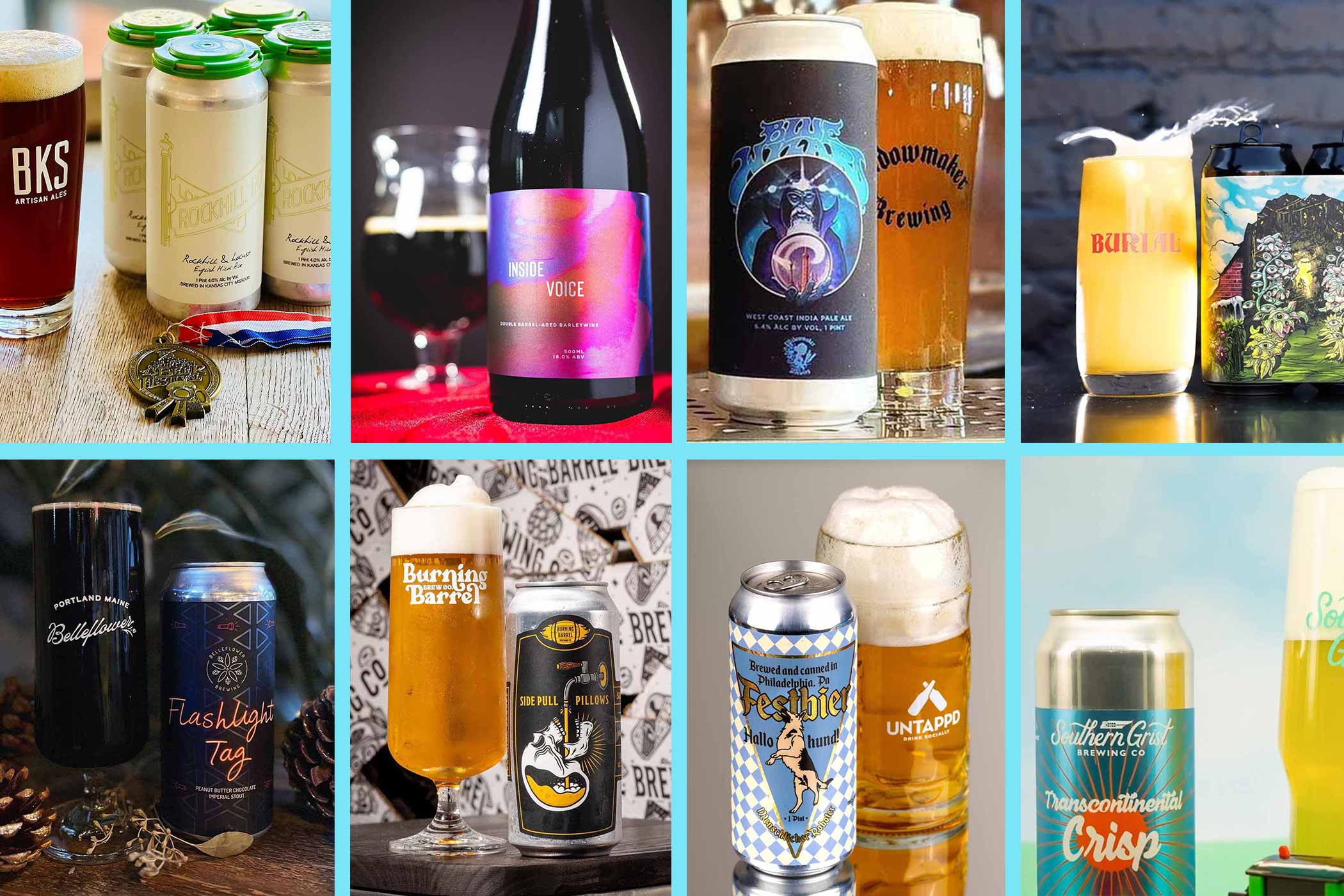The image consists of eight vibrant and colorful rectangular and square pictures arranged in two rows of four, depicting various unique and independent beer and brewery-themed visuals. From top left to right, the first picture shows a glass of brown beer labeled "BKS." Next is an image showing white cans bundled by a green plastic top, with a medal featuring a red, white, and blue ribbon placed in front. The third picture features a bottle with a pink label and an accompanying tulip glass containing a dark liquid. The final image on the top row displays a tall glass with brown beer, featuring foam at the top, next to a can labeled "Burdell," with beer splashing out of the glass.

In the bottom row, starting from the left, the first image shows a dark brew in a tall glass, labeled "Flashlight Tag," beside a can with a dark label with orange writing. The second picture depicts a golden liquid in a glass, labeled "Burning Barrel," with the can suggesting an intricate design resembling intestines. The third picture features a glass with a gold liquid and foam, next to a can illustrating a German shepherd standing on its hind legs. A blue label reads "Fizz Beer." Lastly, the bottom right image contains a glass with a yellowish liquid and foam next to a can from the "Southern Grist Brewing Company," marked with the word "Crisp." The images are rich with hues of yellow, green, brown, dark grays, and blacks, creating a diverse and detailed visual narrative.